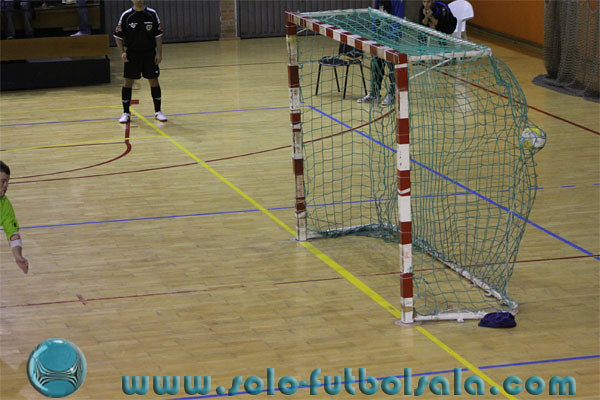In this detailed photograph taken inside a gymnasium, the setting features a light wooden floor marked with various painted lines for game boundaries. Dominating the scene is a rectangular goal similar to a hockey goal, with a striped red and white metal frame and a blue mesh net. A white circular ball has been thrown or kicked into the net, captured mid-flight and pushing the net backwards. There are two visible individuals; one in the background wearing black athletic attire—black shirt, shorts, high socks, and white tennis shoes—looking at the net, and another to the left in a yellow outfit extending their arm forward. At the bottom of the image, there is a logo of a blue soccer ball next to the text "www.solofootballsala.com" in blue lettering, indicating that this is likely an indoor soccer game in progress.